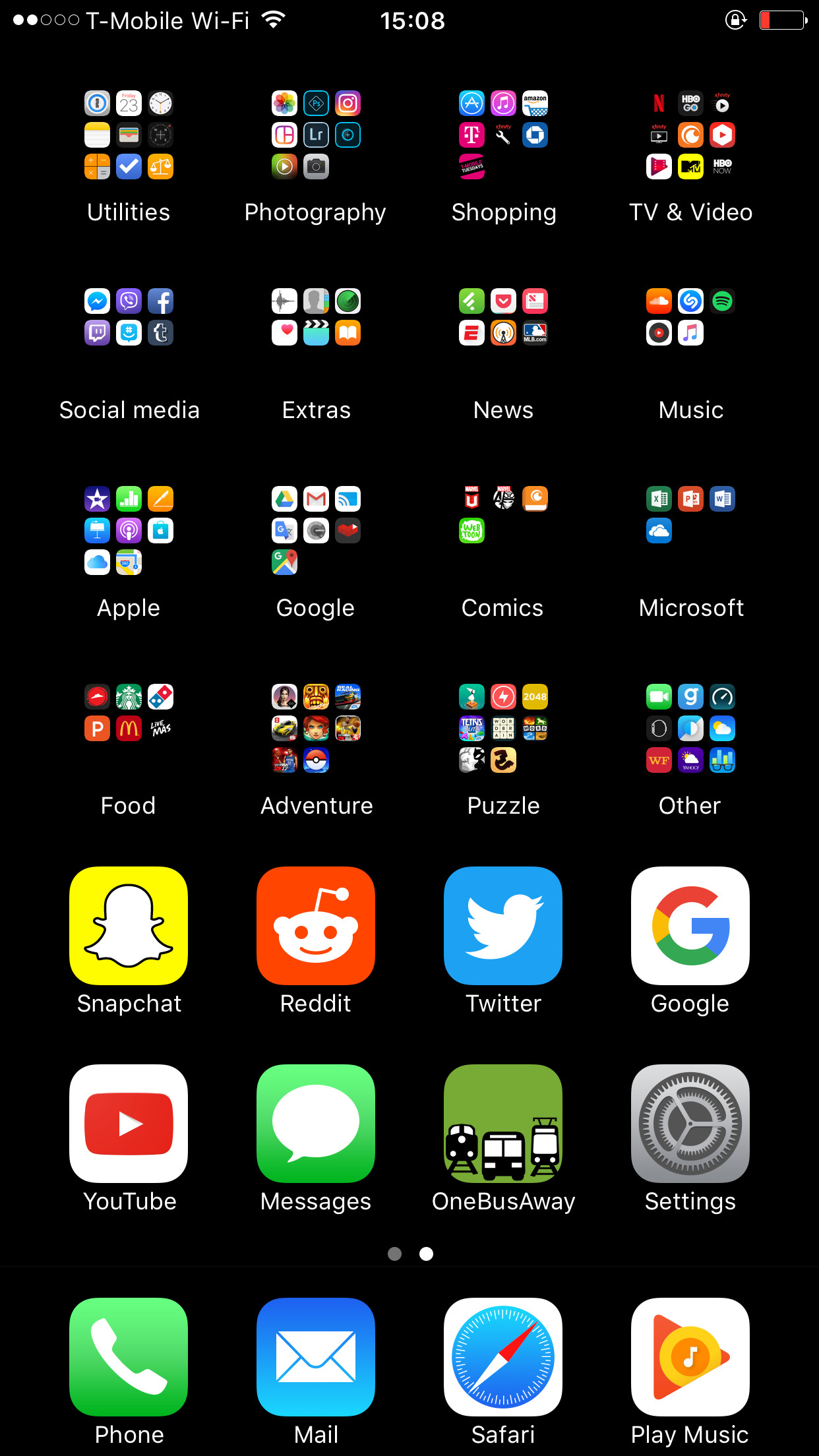The image depicts a smartphone screen with a long, rectangular, vertical black background. At the top of the screen, the status bar shows "T-Mobile Wi-Fi," indicating the network connection, along with the time displayed as "15:08" and a battery symbol with one bar of charge. Below the status bar, the screen is organized into two main sections: app folders and individual app icons.

The upper section consists of four rows of folders, each containing four folders. These folders are categorized and titled accordingly, though the titles are not explicitly mentioned.

The lower section contains three rows of individual app icons. The first row features, from left to right, Snapchat, Reddit, Twitter, and Google. The second row shows YouTube, Messages, One Bus Away, and Settings. The third and bottom row displays the icons for Phone, Mail, Safari, and Play Music, lined up sequentially.

The layout is neat and systematic, providing easy access to both categorized folders and frequently used apps.